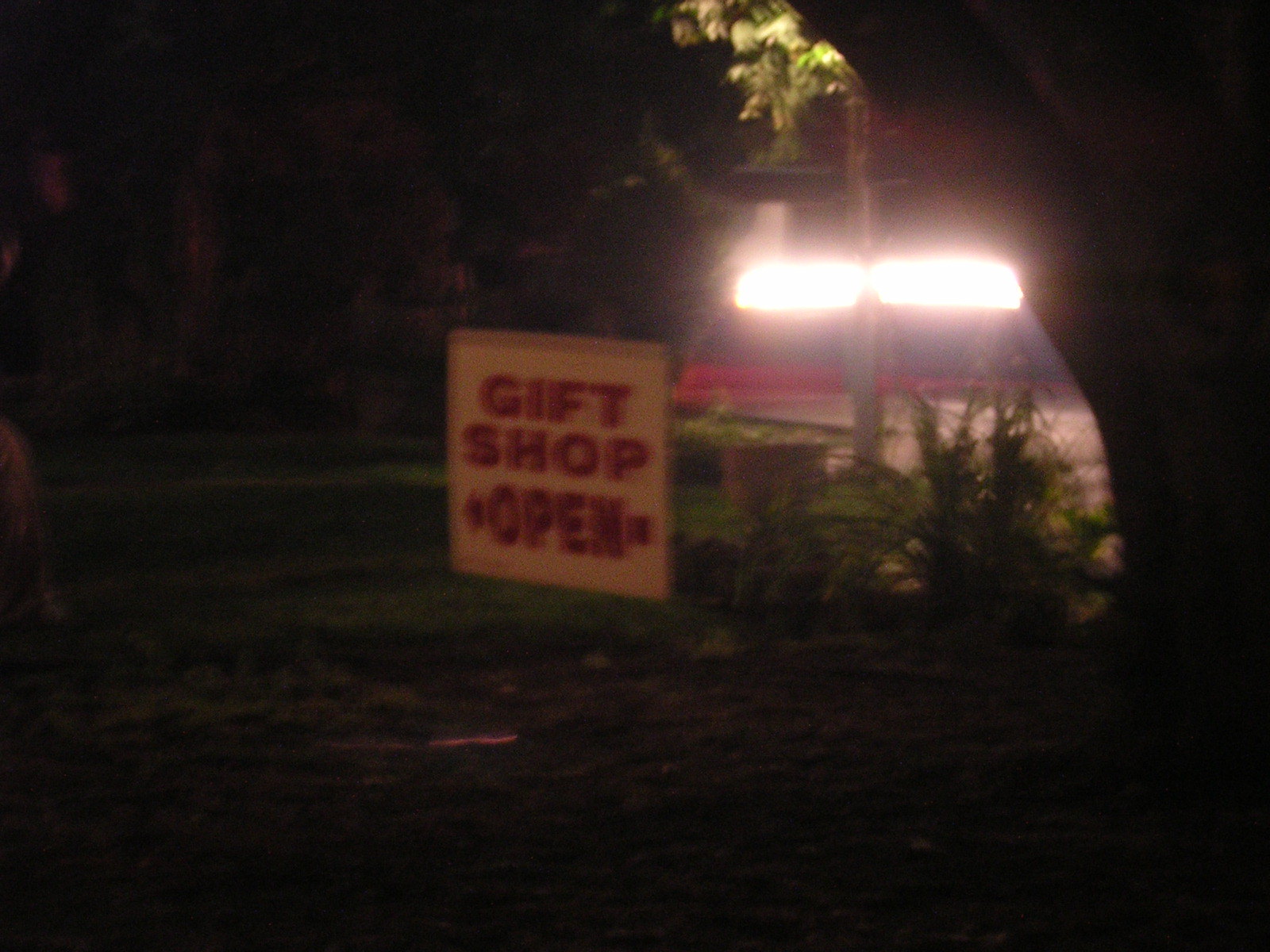A grainy and blurry nighttime photograph taken from inside a car features a vividly lit gift shop sign with red lettering on a white background, proclaiming "Gift Shop Open" with an arrow pointing to the left. The sign is prominently illuminated by two bright, incandescent floodlights above it, creating stark contrasts with the surrounding darkness. Small green bushes and some sparse shrubbery are visible around the sign, hinting at a verdant setting, possibly near a forest or a tourist area. In the background, faint outlines suggest a parking lot, but details are obscured by the pitch-black surroundings and the low-quality exposure of the image. The overall impression is of a lone, inviting outpost amidst an otherwise obscured and shadowy environment.